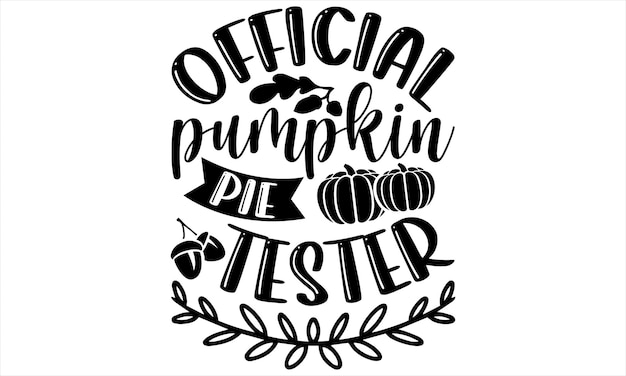The image displays a decorative text arrangement on a white background, with all text and design elements rendered in black. At the top, the word "Official" is prominently arced. Below it, the word "Pumpkin" is written in cursive, with a small black leaf-like structure placed above the 'M' and 'P'. Underneath "Pumpkin," there is a black ribbon-like banner featuring the word "Pie" in white text. To the right of this banner, two black pumpkins with white detailing are situated side by side. Flanking the word "Tester" at the bottom, which is in curved text, are two small icons resembling acorns on the left. At the very bottom of the image, a twig adorned with small laurel leaves adds a finishing touch, arching gracefully from left to right. Surrounding the entire arrangement is a very faint horizontal rectangle outline, framing the central text and decorations.